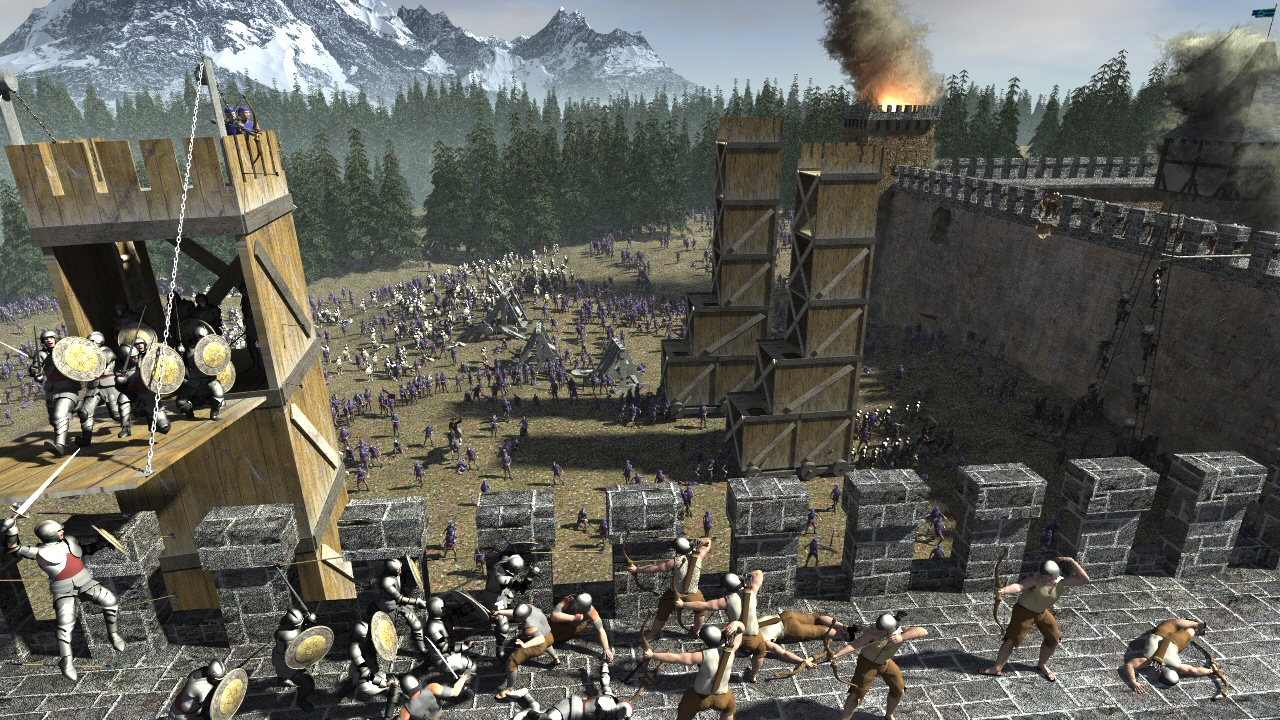The image is a detailed 3D illustration of a medieval battle focused on a siege of a fortified castle. The perspective is from above the massive, solid walls of the castle, where armed soldiers are engaged in combat. Some soldiers are armed with swords and shields, while others are using bows and arrows, with some hiding behind pillars for cover. Below the walls, a large army dressed in blue and white surrounds the castle, with tents scattered across the battlefield. Siege towers and ladders are positioned against the walls, one of which has made contact, allowing attackers to ascend. In this fierce battle scene, there is smoke in the air from fires burning in some of the towers. The background features evergreen trees and majestic mountains with snow-capped peaks, adding depth to the dramatic and chaotic scene.